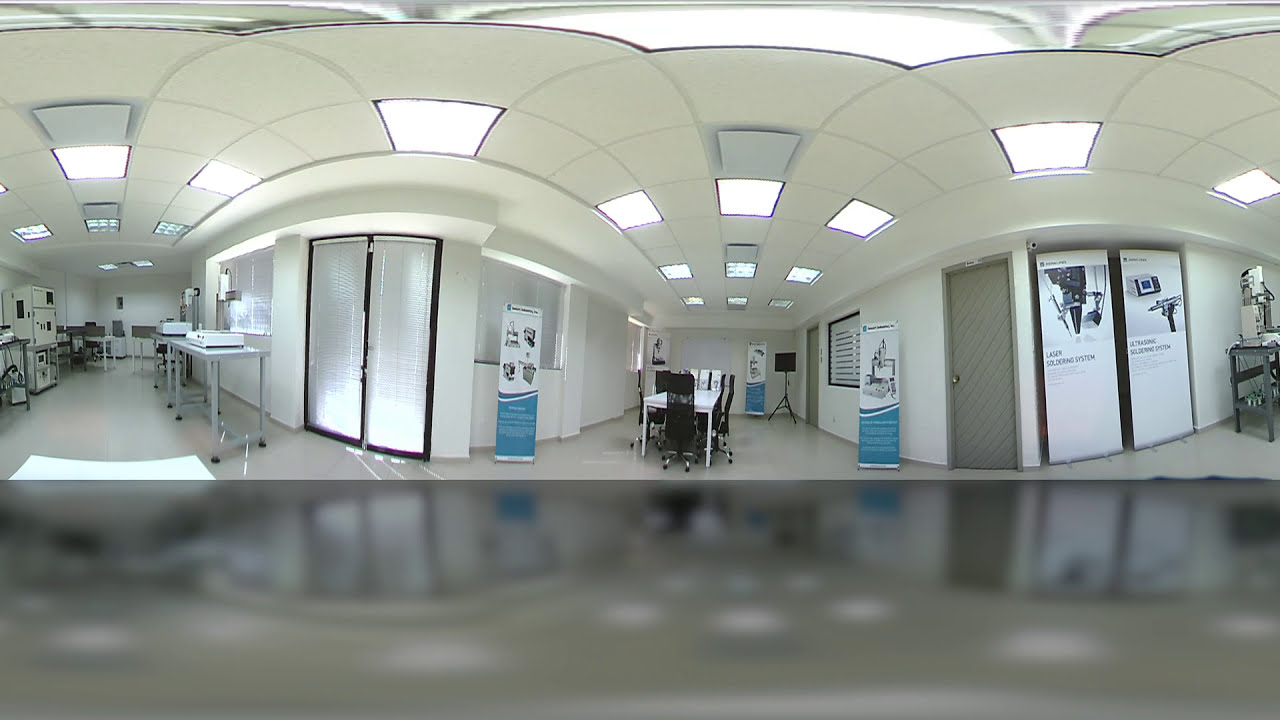The photograph captures a sterile, brightly-lit medical office space, possibly a hospital ward or doctor’s office. The ceiling, comprised of white tiles, features built-in square fluorescent lights and small gray speakers. The walls are primarily white, with white and turquoise signage sprinkled throughout, which includes vertical cardboard billboards likely aimed at visitors. Furniture in the room includes a central white table surrounded by black chairs and several gray, metal equipment stands with white objects on top, suggesting medical supplies. A gray door with a handle is visible, and there appears to be a black monitor or screen positioned at the back of the room. Additional features include off-white medical equipment, a few rolling tables with more medical devices, and windows with white blinds drawn. The overall atmosphere is very clean and orderly, free of any people, reinforcing the sanitary, antiseptic nature of the space. The floor is a white-ish ceramic tile, enhancing the bright, hygienic feel of the room.